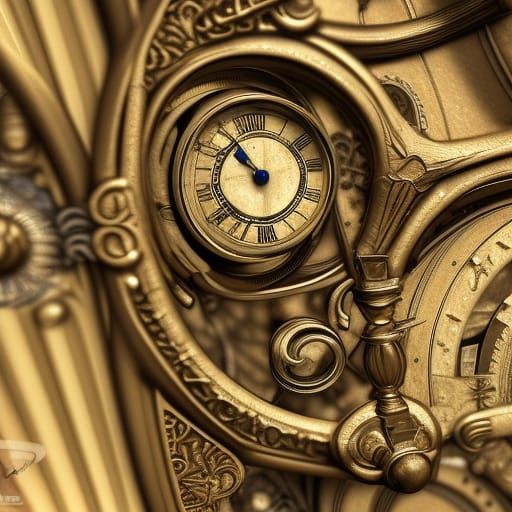The image is a detailed close-up of a small, ornate clock embellished with complex, gold, and bronze-hued decorative elements. The clock, centered in the image, features a light tan face with black Roman numerals and black hands, indicating the time as five minutes to twelve. Surrounding the clock are intricately carved sculptures with various textures, curves, vertical lines, and inlaid details that give the impression of an elaborate metallic structure, possibly part of a larger object. The background is slightly blurred on the left, suggesting depth and focus on the clock and its immediate surroundings. Additionally, hints of another circular object and a handle can be seen, contributing to the complexity and antiquity of the design, which resembles an old-time mechanical contraption or an ancient decorative artifact.